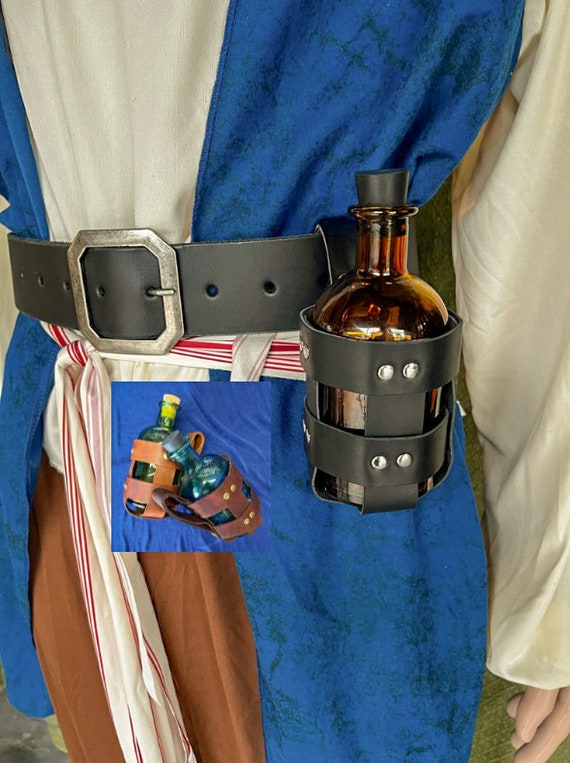The image depicts the midsection of a mannequin adorned in a blue smock reminiscent of pirate attire, layered over what appears to be a white shirt. The mannequin is easily identifiable due to its plastic hands. A standout feature is the black leather belt cinched around its waist, equipped with a prominent silver buckle. Tied around the mannequin’s middle is a red and white scarf, adding to its vintage ensemble. Attached to the belt is a black leather water bottle holder embellished with six silver rivets, which cradles a brown glass bottle sealed with a cork. Additionally, there are two unattached bottles in the scene—a yellow one and a blue one—suggesting different variations of the carrier, possibly indicating an advertisement for the carrying device. The figure also sports white cream-colored sleeves peeking from beneath the smock, enhancing the historical feel of the outfit. The background and overall composition indicate that the image was digitally created, focusing on medieval or old-fashioned themes.